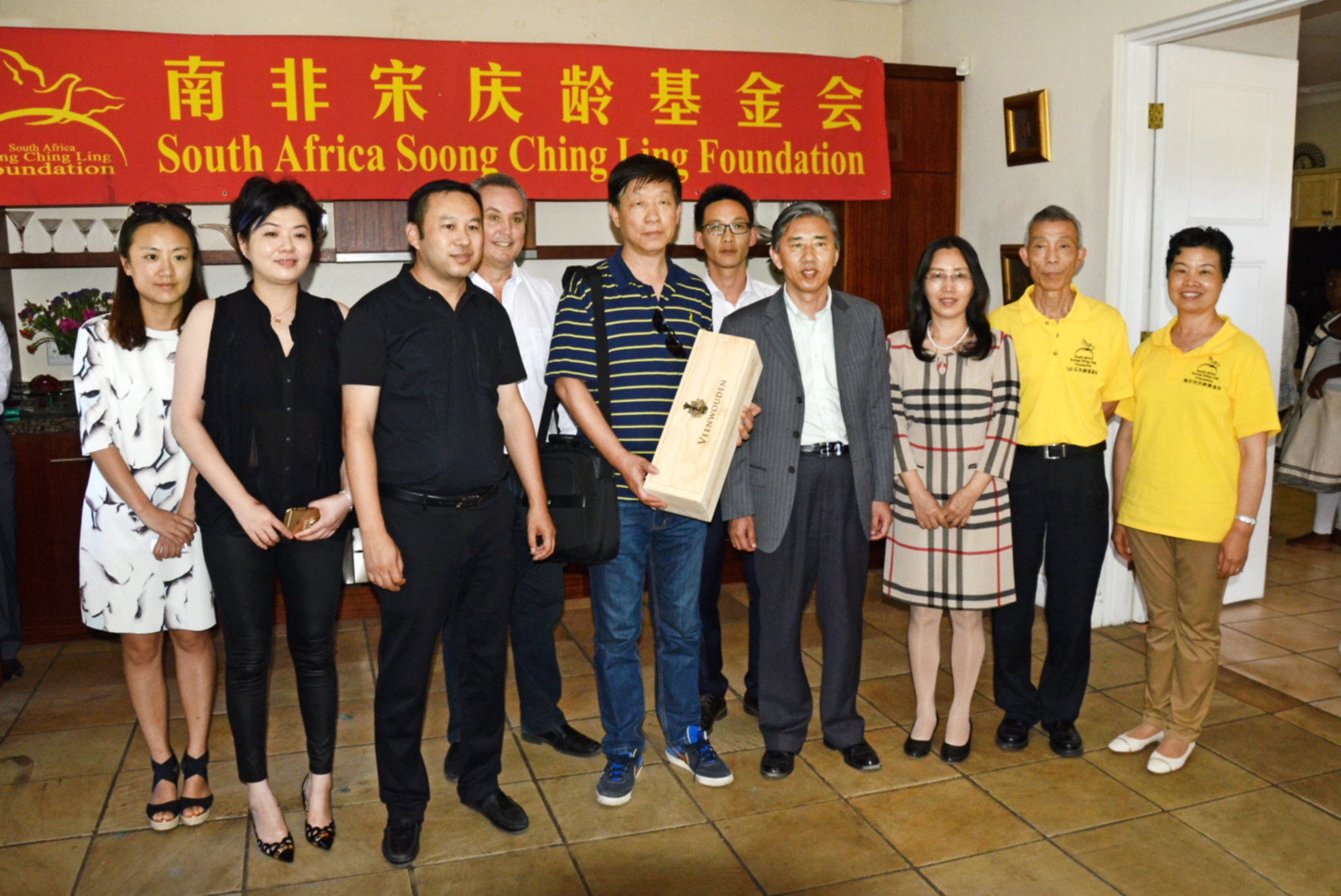A diverse group of approximately 10 to 11 people, the majority of whom appear to be Chinese, are gathered for what seems to be a formal photograph. The backdrop is a prominent red banner with yellow text written in Chinese, with an English translation below that reads, "South Africa Song Ching Ling Foundation." The group includes three to four women and six men. The women are dressed in a variety of outfits including dresses, blouses, and knee-length shorts. The men are dressed in attire ranging from yellow t-shirts with logos, to a black shirt with black pants, a gray suit, a striped pullover, and blue jeans. The gentleman in the center, who stands out, is holding a wooden box labeled "Wien Wooden," which resembles a container for whiskey or wine, possibly an award. The arrangement suggests a celebratory or commemorative event, likely associated with the foundation mentioned on the banner.